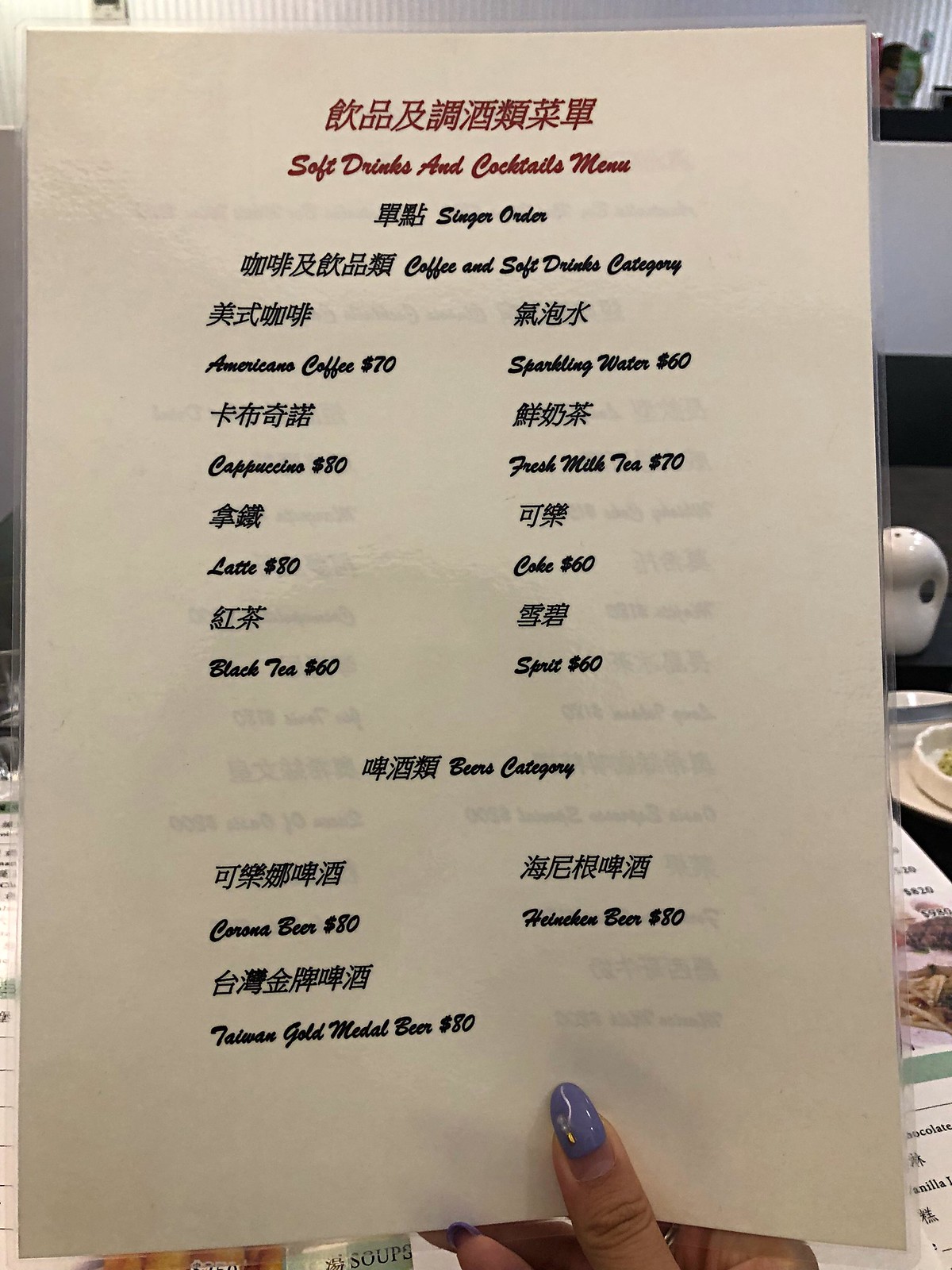The image depicts a laminated menu held by a woman with light lavender nail polish, visible on her thumbnail and the tip of her pinky at the bottom right corner of the menu. The menu is printed on a single white sheet encased in clear plastic, with red kanji characters at the top. Below the kanji, the text "Soft Drinks and Cocktails Menu" is displayed in English. The menu features items listed in both an Asian language and English, with smaller, harder-to-read subtext stating "coffee and soft drinks company." The layout includes dual columns with prices and a brief pause between the sections, followed by another set of double lines. In the background, a table adorned with additional menus and round white plates is visible, set against an off-white wall.